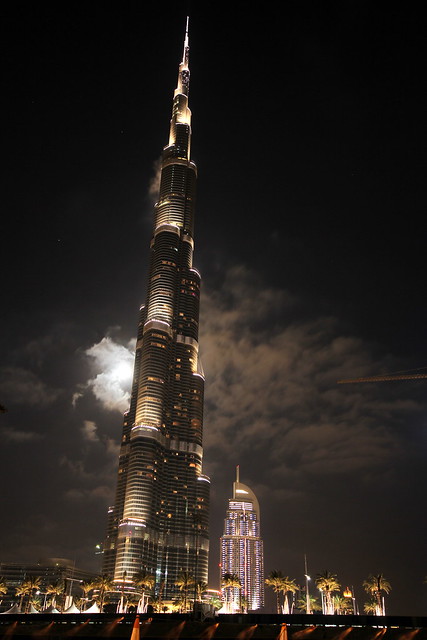This vertical nighttime photograph captures a striking cityscape dominated by an exceptionally tall, futuristic skyscraper that stretches skyward like an upside-down ice cream cone or needle, accentuated by its pointed top. The sky is almost completely black, emphasizing that it is taken at night, save for the moon shining brightly through wisps of clouds near the center of the image, which adds an ethereal glow to the scene. The skyscraper, adorned with numerous lights and windows, emits a majestic and incredible aura, with its rounded, tapering structure stacking narrower sections one on top of the other as it ascends. Beneath this architectural marvel, significantly shorter structures with blue lights and palm trees softly illuminated by the urban glow punctuate the lower portion of the image, providing contrast and enhancing the skyscraper's towering presence.